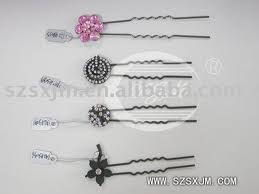The photograph, set against a grey background, showcases four ornately designed bobby pins laid on their side, with the decorative ends on the left and the open ends on the right. A prominent watermark across the center reads "Alibaba.com," and another in the bottom right corner states "www.szsxjm.com." Each bobby pin features a price tag hanging to the left. The topmost bobby pin boasts a pink shiny crystal arrangement resembling a flower. Below it, the second pin displays a bull's-eye pattern of alternating white rhinestones and black circles. The third pin features a simple black circular design adorned with white dots. The bottom pin is a five-petal black flower with a rhinestone center. The black bobby pins themselves have classic wavy sections. In summary, the photograph is a detailed product image designed to present the intricate beauty of these decorative hair accessories.